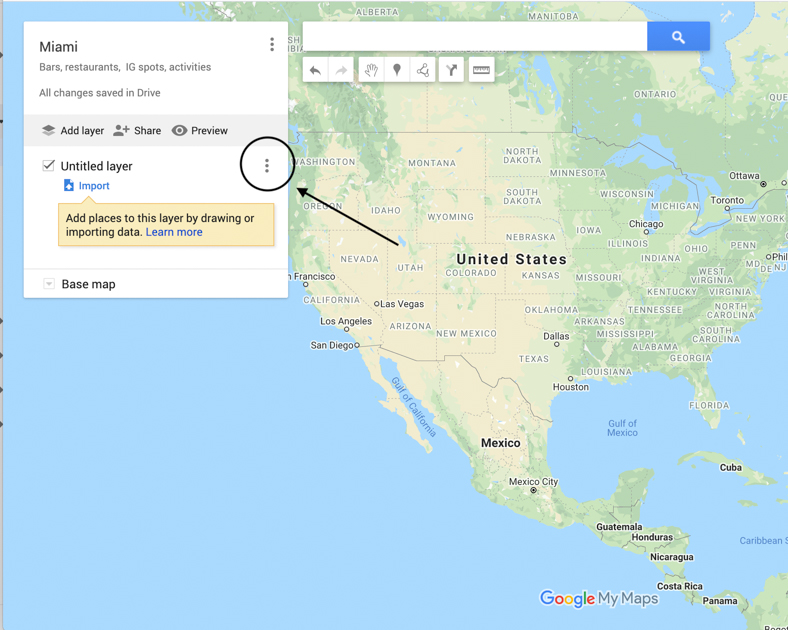This detailed caption describes a digitally annotated map of North America with a particular focus on the United States and additional features including various tools and icons for customization:

>>> 
"A detailed screenshot of a digital map of North America, prominently featuring the United States while also including Canada, Mexico, Central America, and parts of the Caribbean. At the top of the image, a search bar with a blue search button accompanies icons representing webpage customization options. Towards the top left, a floating chart is titled 'Miami' and includes clickable options labeled 'Bars', 'Restaurants', 'IG Sports', and 'Activities'. Just below this chart, the text 'All changes saved in Drive' is visible. 

A gray banner underneath the chart showcases three icons: 'Add Layer', 'Share', and 'Preview'. A checked box marked 'Untitled Layer' lies just below this banner, next to an 'Important' tag with a talk bubble. The talk bubble, set against an orange background, reads 'Add places to this layer by drawing or importing data' in black text. 

Further annotations include a circle around three vertical dotted lines beside the 'Untitled Layer' text, highlighted by a black arrow stemming from the state of Utah. The bottom of the map is labeled with 'Base Map', and a 'Google My Maps' logo is located at the bottom right corner of the image."
<<<